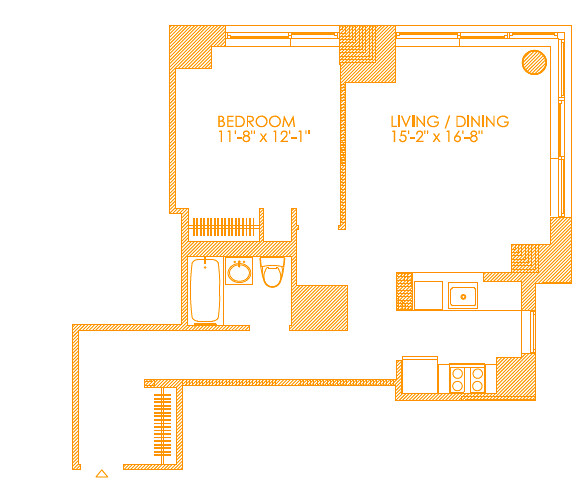This top-down view of an apartment floor plan reveals a detailed layout of the living space. At the center, the largest area is designated as the living/dining room, measuring 15 feet 2 inches by 16 feet 8 inches. The right-hand corner of this room is suitable for placing a dining table, while the remaining space is open. 

Adjacent to the living/dining room on the left, a partition separates the area into a bedroom highlighted in orange lettering. The bedroom measures 11 feet 8 inches by 12 feet 1 inch and includes a closet and a doorway for easy access.

Below the bedroom, a small bathroom is enclosed, featuring essential fixtures such as a toilet, sink, and bathtub. To the immediate right of the bathroom, a hallway provides access to various parts of the apartment.

This hallway leads directly to a compact kitchen located on the right, equipped with spaces for a sink, refrigerator, and a small oven. Additionally, to the left of the hallway near the entrance, there is another hallway leading to the front door of the apartment, with a closet area to the right for extra storage.